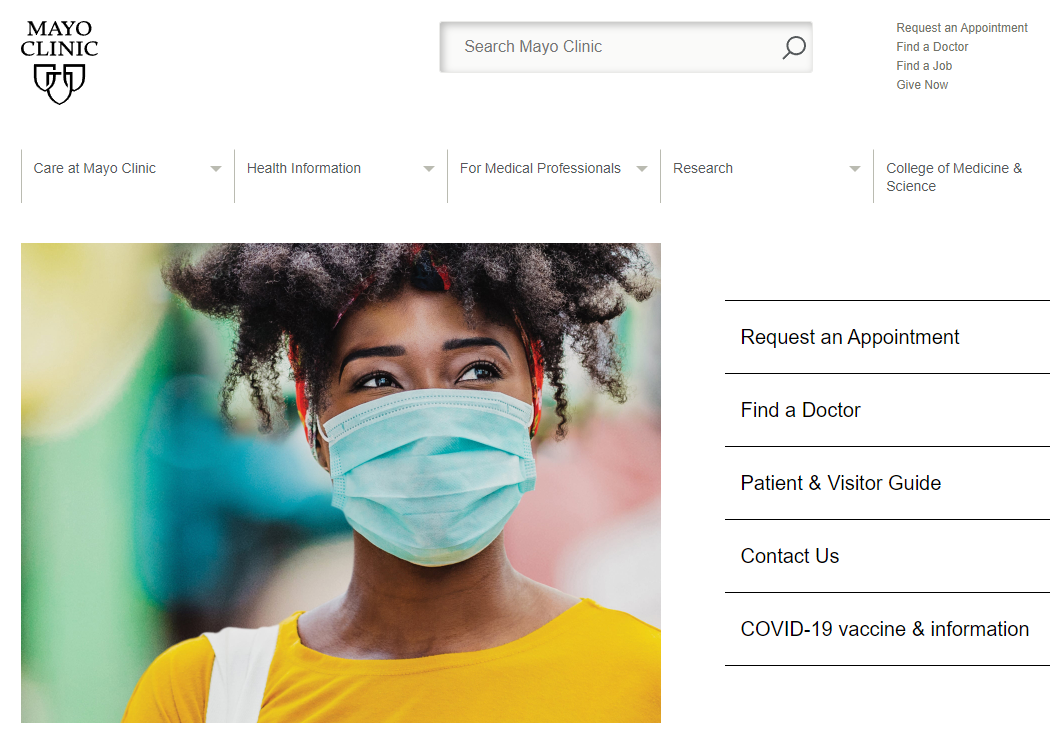The image is a screenshot of a webpage from the Mayo Clinic. At the top left, the logo "Mayo Clinic" is prominently displayed. In the top center, a search bar with the placeholder text "Search Mayo Clinic" is visible. On the top right, several navigation options are listed: "Request an Appointment," "Find a Doctor," "Find a Job," and "Give Now."

Below this header, there are five primary tabs arranged horizontally from left to right: "Care at Mayo Clinic," "Health Information," "For Medical Professionals," "Research," and "College of Medicine and Science."

Further down the page, there are additional sections listed vertically: "Request an Appointment," "Find a Doctor," "Patient and Visitor Guide," "Contact Us," and "COVID-19 Vaccine and Information."

On the left side of the image, there is a photograph of a person with the following features: she has black hair, black eyebrows, black eyes, and is wearing a yellow top. She is also wearing a face mask and is carrying a white strap over her shoulder.